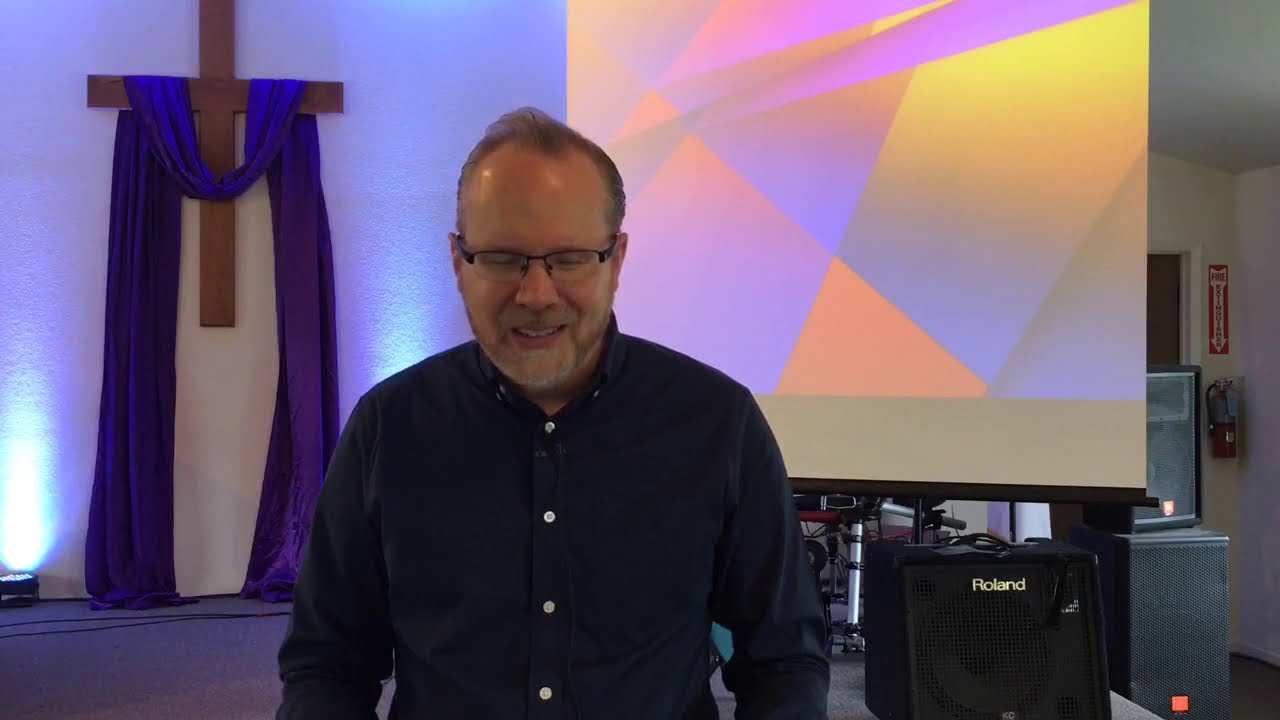In this horizontal rectangular image, a middle-aged white man stands at the center. He is facing forward but looking down, speaking with his mouth open, revealing his teeth. He wears glasses and sports a receding hairline with combed-back brown hair, and a sparse beard and mustache with shades of white and brown. He is dressed in a long-sleeved, dark navy blue or possibly black button-down shirt with white buttons.

The background indicates the interior of a Christian church. Behind the man, slightly to his right (our left), a wooden cross hangs on the wall, draped with a purple or blue velvety fabric. To his left (our right) a black Roland speaker bag with white print lies on the floor. Directly behind him, a large projector screen displays abstract geometric shapes in various colors. The floor is gray, with wires running across the lower right-hand corner of the image. Additional white walls and a door are visible behind the projector screen, and lights are positioned on the floor near the cross, casting dim light across the scene.